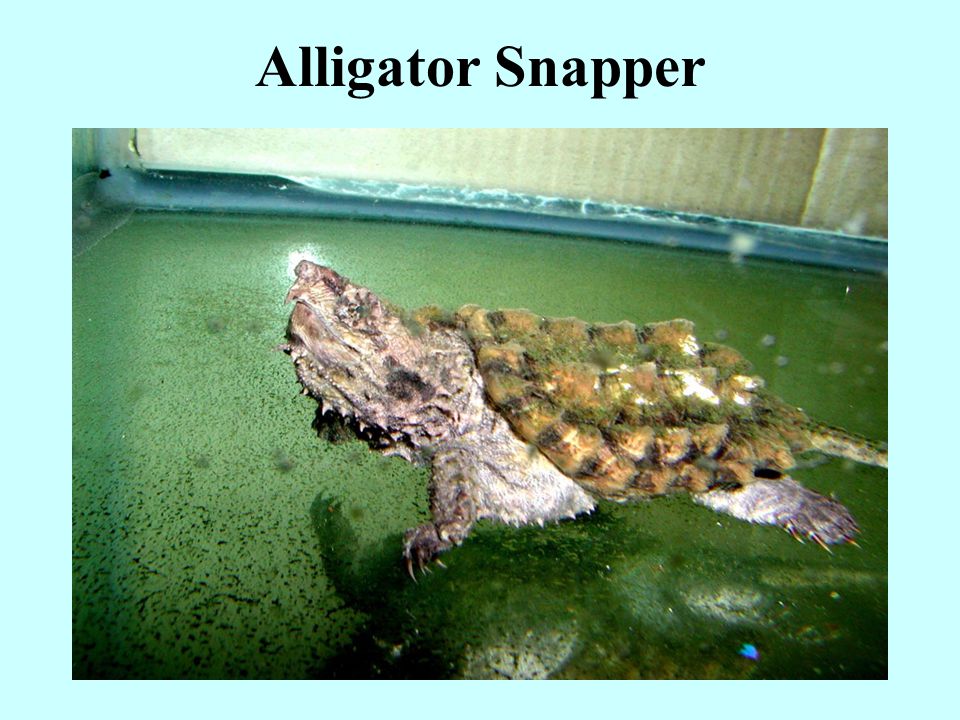The photograph titled "Alligator Snapper," framed by a light blue border, depicts an alligator snapper in a murky, greenish, swamp-like environment. The words "Alligator Snapper" are prominently displayed at the top in bold Times New Roman font against a turquoise blue background. The image is in landscape orientation and features an old, turtle-like creature with a rugged, patterned shell in shades of beige, dark green, black, and rust. Its body, a dark gray hue, exhibits long, sharp claws on both its arms and legs. The snapper is positioned slightly off-center, swimming from the right toward the left side of the tank, and casting a reflection in the dirty water below. The head, on the left side, is a mass of misshapen, lumpy brown and beige colors, making its facial features indistinguishable. Surrounding the water is a setting that suggests an indoor environment, possibly a tank in a museum or a specialized exhibit, with a cardboard piece in the background likely used to block light.